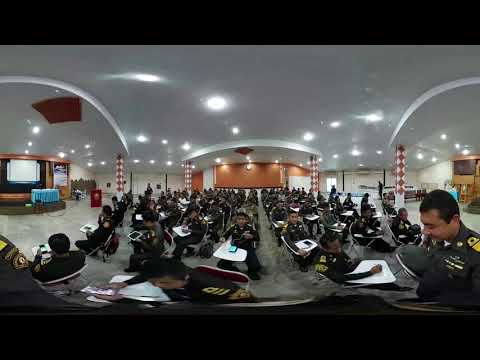In this detailed image, we see a large, well-lit room inside a building, densely populated with around 50 to 60 people seated in rows. The room features numerous fluorescent lights on the ceiling, with red and white decorations adorning some beams and poles throughout. The ceiling is gray with speckles of white dots, accessorized with white arches on the left and right sides. A brown rectangular structure with white arches spans the middle of the ceiling.

Most individuals appear to be in dark-colored military uniforms, though some figures in the background are harder to distinguish. They are seated in rows of mini desks, arranged in a pattern of approximately 10 rows by 20 columns. Their seating seems rather haphazard, with some people facing to the right, others to the left, and still others toward the center—indicating there might be multiple instructors or speakers present. 

A man in uniform stands to the right, looking down, perhaps reading something or preparing to address the group. Despite the crowded setting, the atmosphere suggests a state of waiting, possibly for an instruction or announcement, in what could be a pre-deployment briefing or a training session. The room itself is clean and well-maintained, with several decorations and monitors visible in the background.